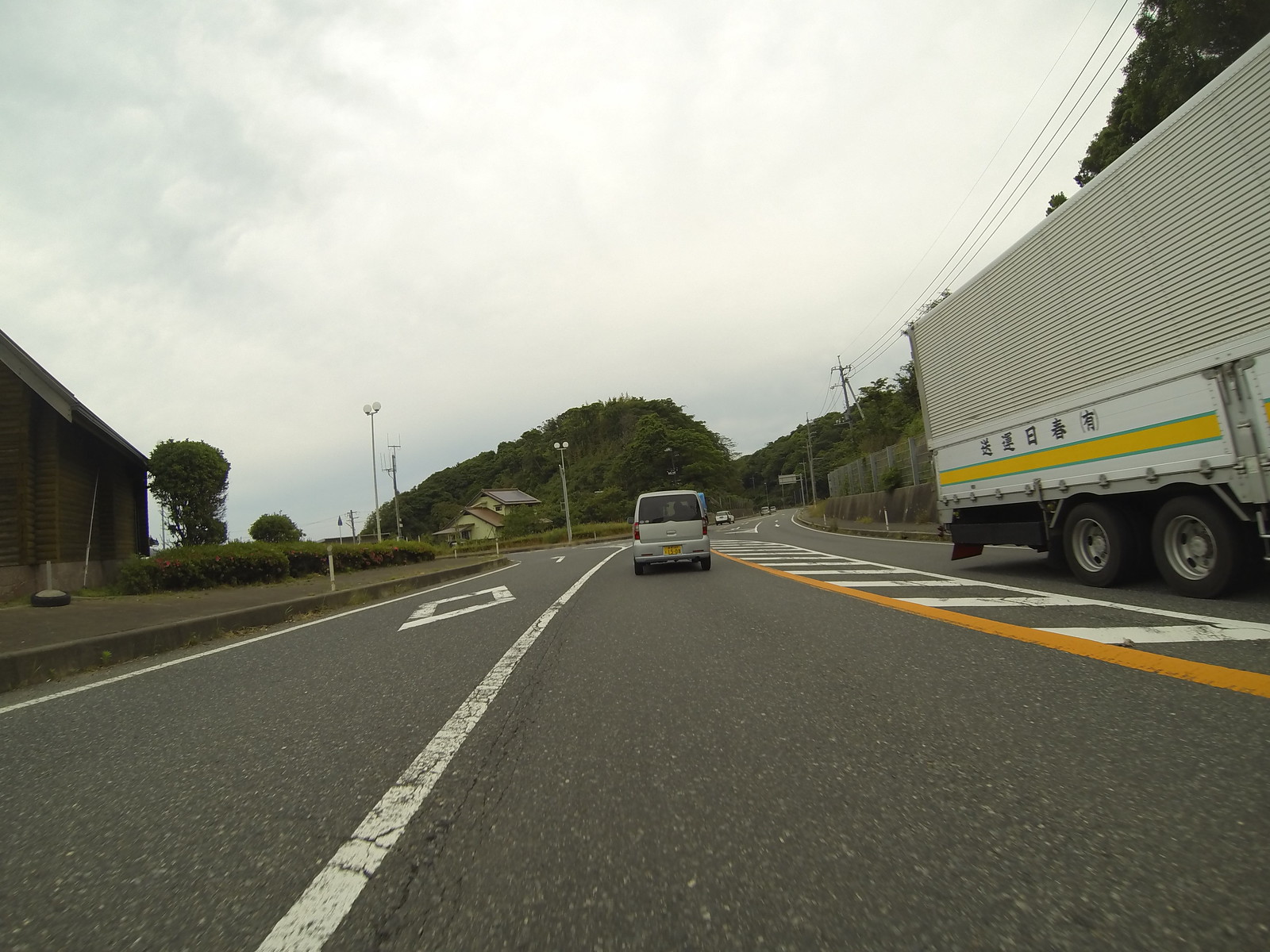The image, captured from a dash cam, shows a stretch of a dark gray freeway. The view focuses on the left lane marked with a distinctive white diamond-shaped pattern, indicating it might be an HOV (High Occupancy Vehicle) lane. Ahead, a silver minivan with darkly tinted rear windows leads the way. To the right, a white semi-truck travels in the opposite direction, showcasing two prominent side wheels and adorned with foreign characters, likely Japanese or Chinese, on its side. The background reveals a verdant hillside adorned with very tall trees, adding a touch of nature to the scene. On the left, a dark brown building stands out. Above, the sky is overcast with light gray clouds, suggesting a potentially overcast day.